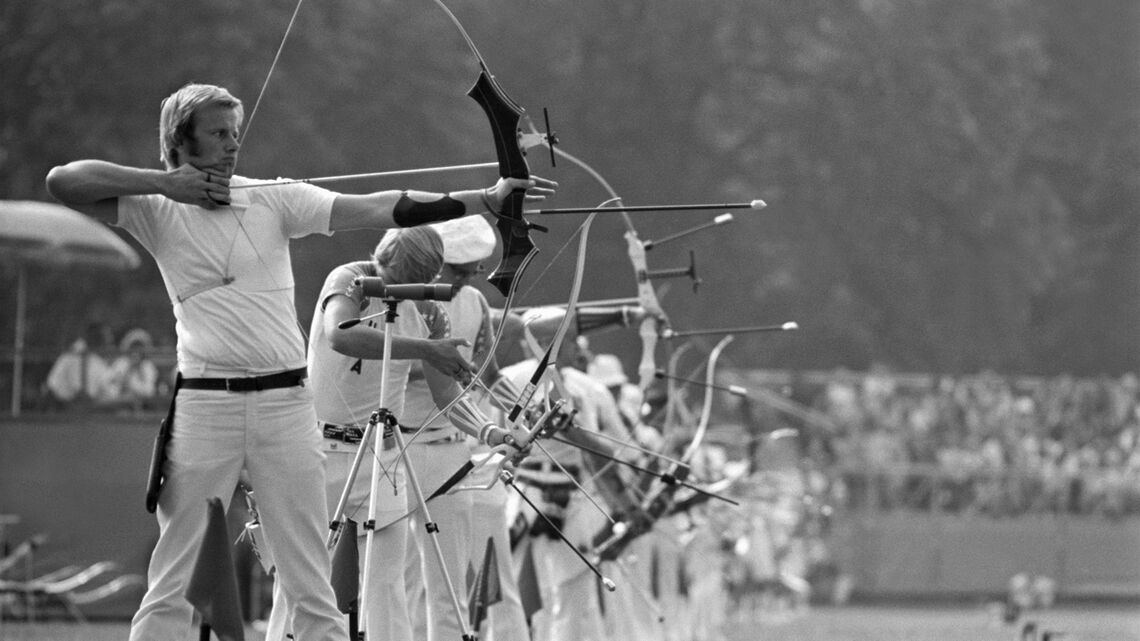This black-and-white photograph captures an intense moment at what appears to be an archery tournament, possibly the Summer Olympics. The image is notably wider than it is tall, emphasizing the long line of archers, approximately 10 to 15, all dressed uniformly in white shirts and pants with black belts. In the foreground, one archer, his face focused and determined, stands poised with his bow drawn back, seconds from releasing his arrow. The other archers are in various stages of preparation, with some stringing their bows and others knocking arrows. The background, blurred but discernible, features a crowd of spectators behind a fenced area, along with visible trees and an umbrella stand. The spectators have a distant, almost ghostly presence due to the blurriness, but their numbers suggest the significance of the event.